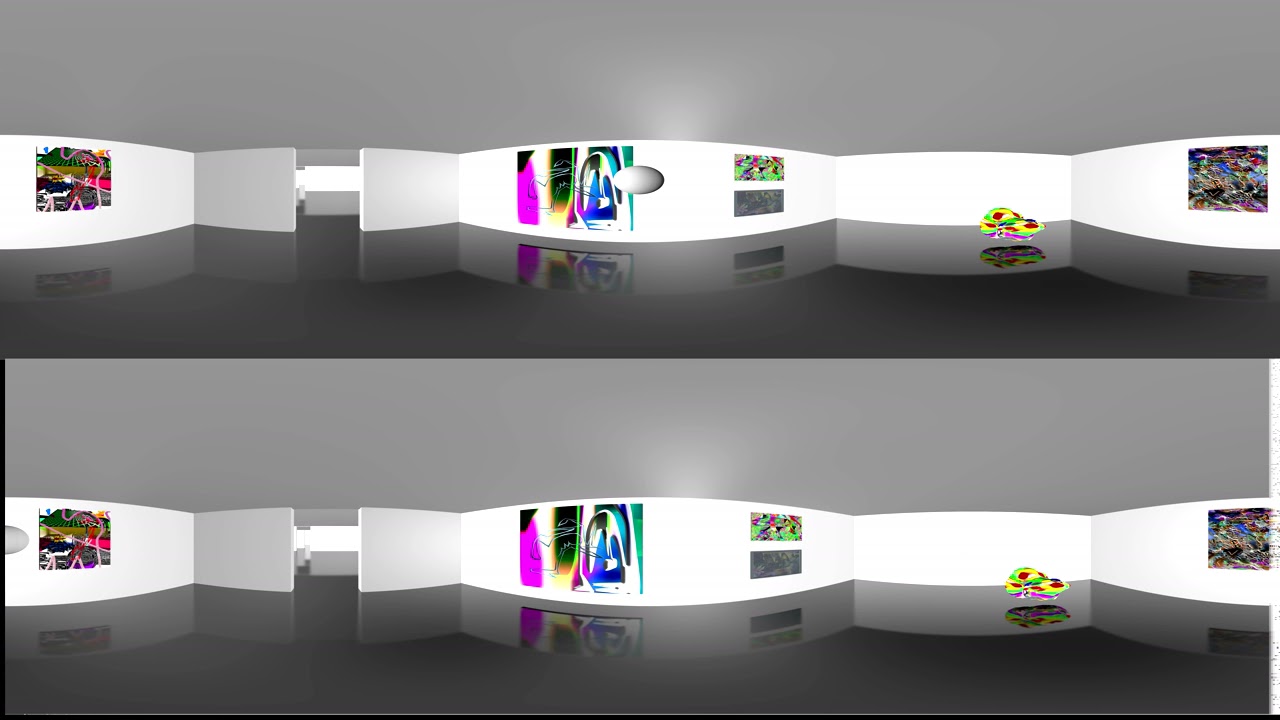The image depicts a digital rendering of an art museum with two almost identical versions presented one above the other. The scene features pristine white walls adorned with various modernistic, multicolored paintings, including hues of pink, blue, and white. The museum space has a dark, reflective floor and a simple gray ceiling. In both renditions, there is a notable white circle—centrally placed between two paintings in the top image and shifted to the far left in the bottom image. The background gray shading varies between the two images, with the top image displaying a gradient from lighter gray at the top to darker gray at the bottom, and the bottom image featuring the reverse. This virtual gallery, likely designed with a computer construction or engineering program, evokes the ambiance of a contemporary art space in a city like New York, inviting viewers to explore its minimalist yet sophisticated environment.